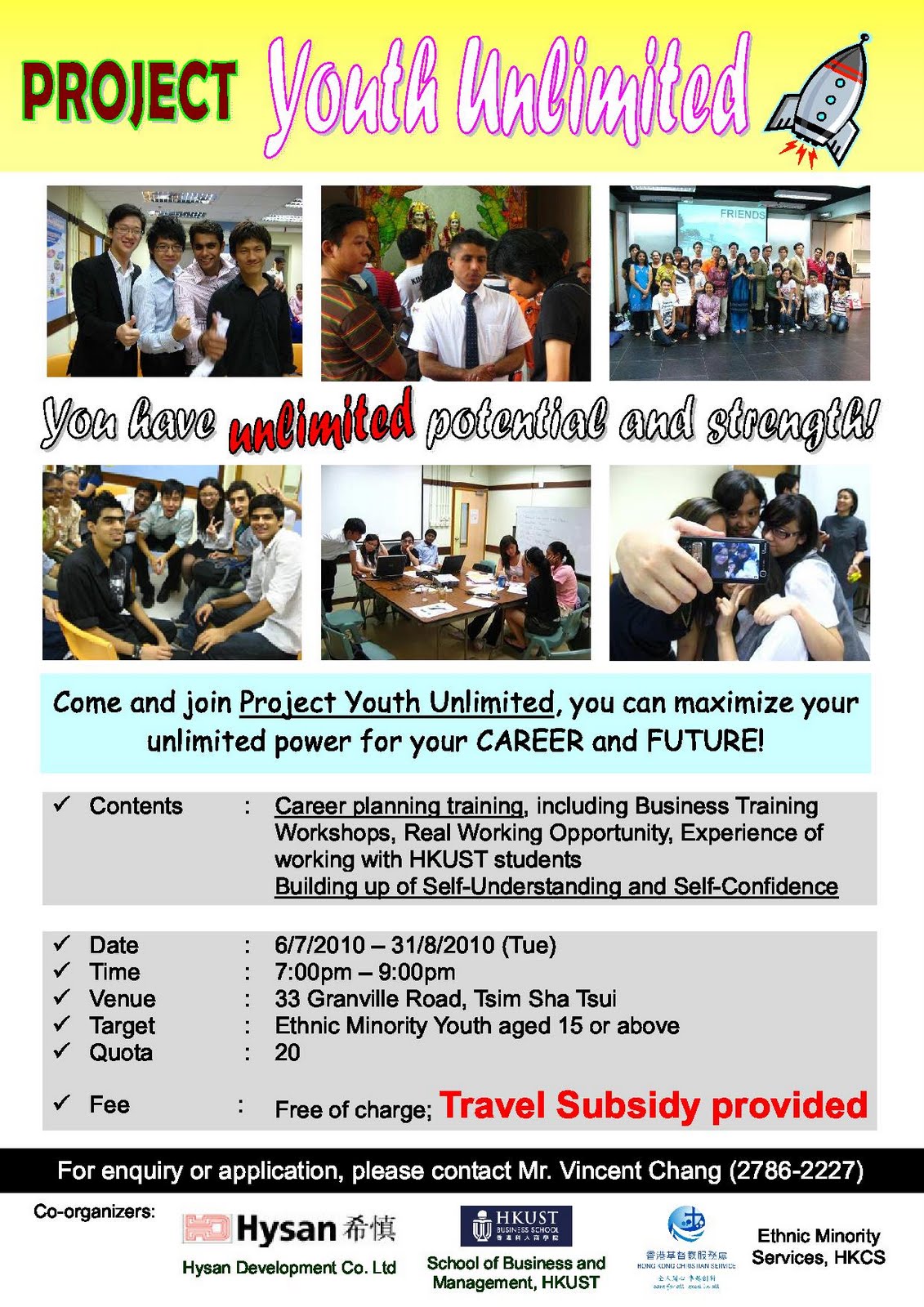This image is a screenshot of a promotional poster titled "Project Youth Unlimited." Dominating the visual space is a striking image of a rocket soaring into the sky, symbolizing boundless potential and aspiration. Beneath the rocket, there are six vibrant photographs showcasing school children who are part of the School of Business and Management (also known as UST), highlighting the program’s active participants and their engagement.

Centrally positioned on the poster is an inspiring slogan: "You have unlimited potential and strength," with the word "unlimited" emphasized in bold red to draw attention. Further down, a notable call-to-action box invites readers to "Come and join Project Youth Unlimited," encouraging them to maximize their potential for future career growth. 

The poster also meticulously lists essential details about the project, including:
- The event contents.
- Time, date, and venue specifics.
- The target audience and quota, specifying that there are 20 available spots.
- An assurance that the participation fee is free of charge.
- Information on a provided travel subsidy for participants. 

For those interested in joining or seeking more information, the poster advises to contact Dr. Vincent Chang, offering his phone number, 2786 2227, for inquiries or applications.